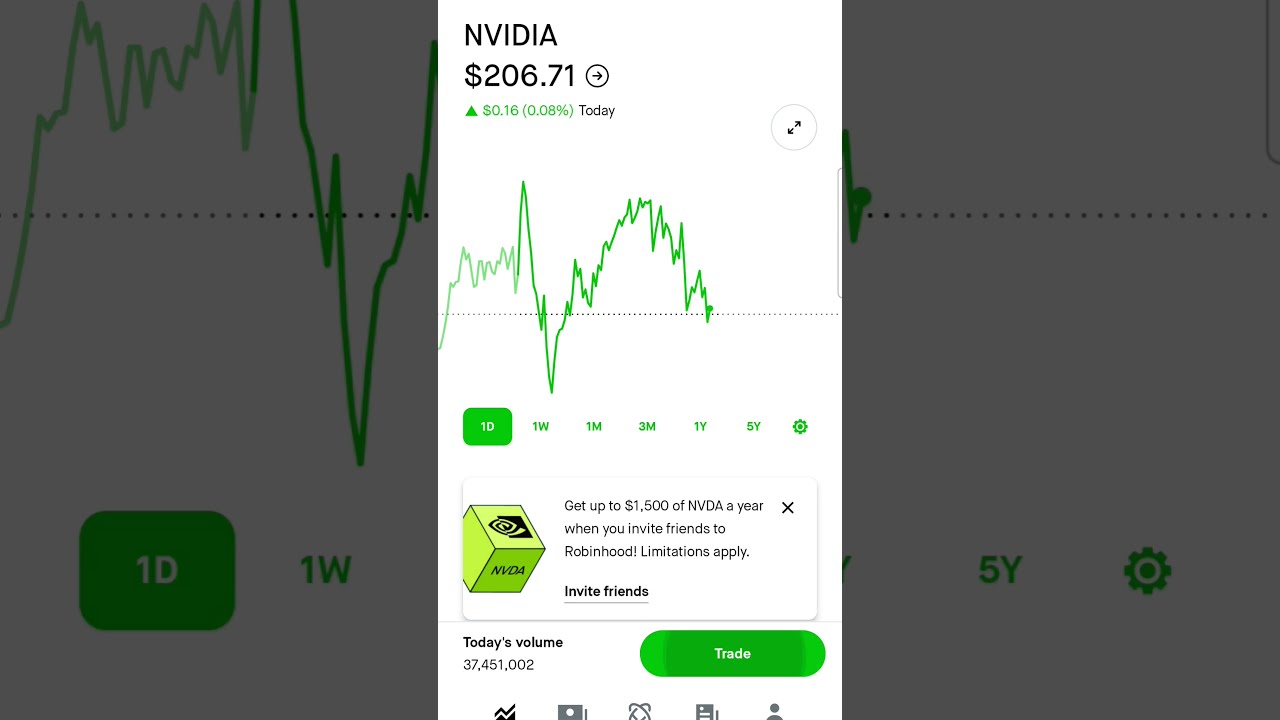The image is a detailed screenshot from an investment app displaying the stock information for NVIDIA. The background is predominantly white with black text and several green elements highlighting key information. At the top, "NVIDIA" is prominently displayed in black, followed by the stock price, which reads $206.71. Below the price, there is a green upward arrow indicating an increase of $0.16, or 0.08% for the day.

In the center of the image, a distinctive green line graph charts the stock's fluctuations, showing its performance over a one-day period. The graph includes the label "1D" in white lettering inside a green square, with additional options for one-week, one-month, three-months, one-year, and five-year views. Additional interface details suggest the ability to trade the stock with a button labeled "Trade."

At the bottom of the image, it's noted that today's trading volume was 37,451,002 shares. Closer inspection reveals a small area mentioning an offer: "Get up to $1,500 of NVIDIA a year when you invite friends to Robinhood. Limitations apply." The screenshot also includes navigational elements and informational buttons under the graph, with one prominently marked as "Transfer" in green, indicating a clickable button. Overall, the image provides a comprehensive snapshot of NVIDIA's stock performance within the app's interface.